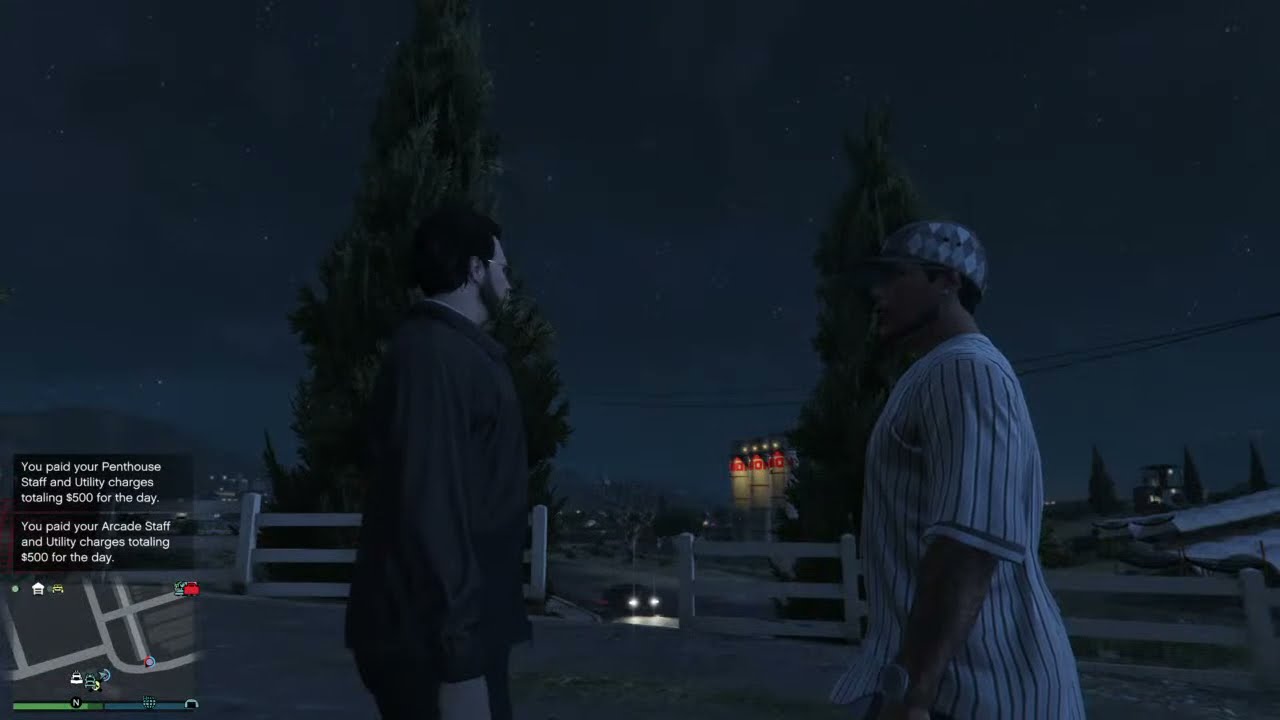The image is a screenshot from a GTA-style video game, taken during nighttime under a star-filled sky. In the center of a road, two characters face each other. The character on the left, a white man with a dark beard and possibly wearing glasses, is dressed in a black suit. The character on the right, a black man, wears a white tunic with black or gray stripes and a gray and white diamond-pattern ball cap. The roadside is lined with wooden fences, and in the background, two tall fir trees stand prominently. Below the trees, another road and some buildings are visible. Additional details in the scene include a car approaching in the background and a lit-up sign with yellow lights. In the bottom left corner of the screen, a map is visible above white text on a black background that reads: "You paid your penthouse staff and utility charges totaling $500 for the day. You paid your arcade staff and utility charges totaling $500 for the day."